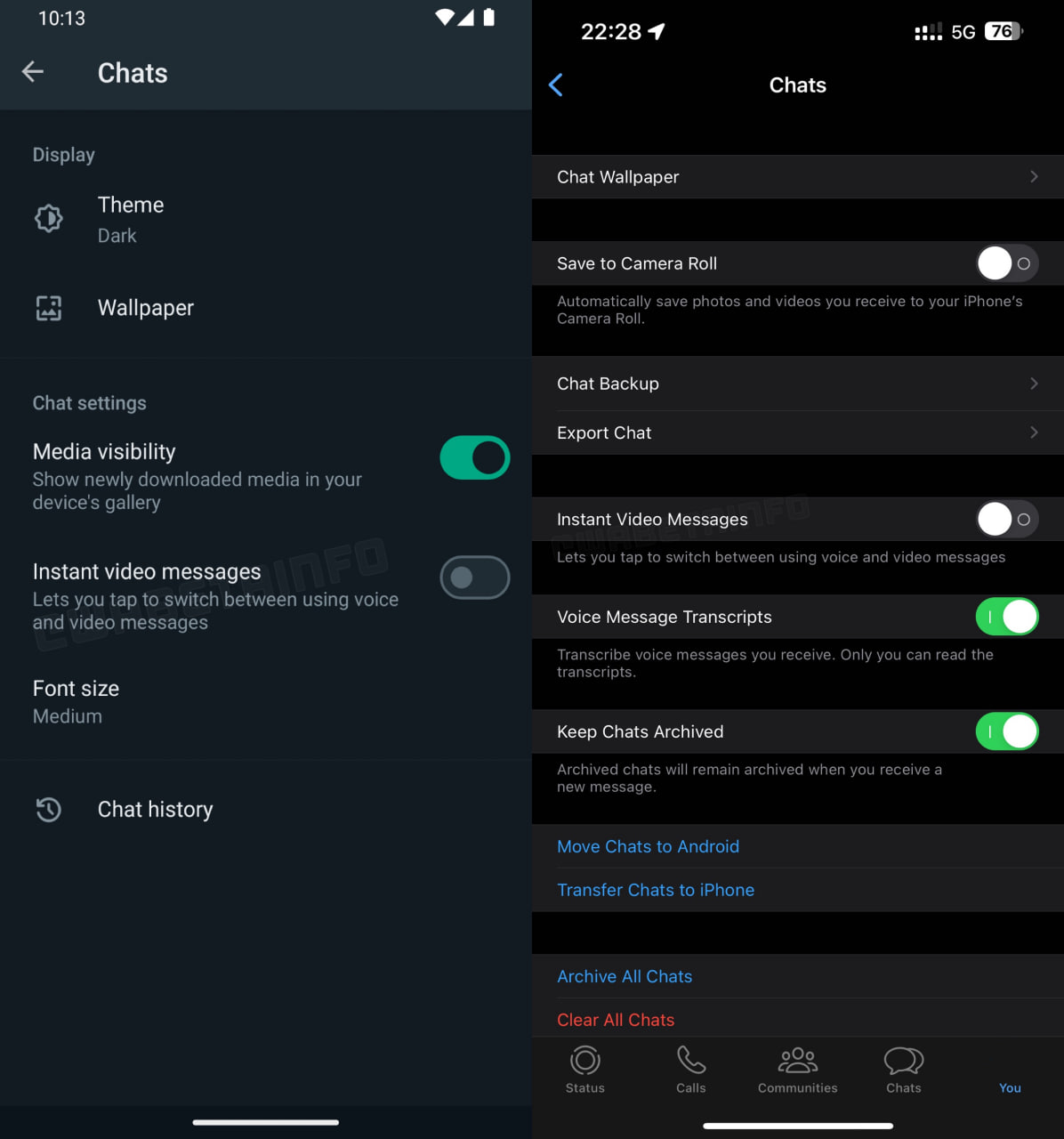The image appears to be a composite of two vertically aligned screenshots from a smartphone. 

On the right side of the split image, the top-right corner displays the phone's battery icon indicating a 76% charge, followed by a "5G" network status, and a signal strength icon showing two bars. The top-left corner shows the time as 22:28. Centered at the top, the word "Chats" is prominently displayed.

Directly below "Chats," there is a list of options in a cascading order: 
1. Chat Wallpaper
2. Save to Camera Roll
3. Chat Backup
4. Export Chat
5. Instant Video Messages
6. Voice Messages
7. Transcripts
8. Keep Chats Archived

At the bottom of this list, written in blue, are options for:
- Move Chats to Android
- Transfer Chats to iPhone
- Archive All Chats

Finally, in red writing at the very bottom, it says:
- Clear All Chats

The bottom section of the right image features four icons representing various functions:
1. Status (depicted by a circular icon)
2. Calls (shown with a phone icon)
3. Communities (represented by an icon of multiple people)
4. Chat (indicated by a chat bubble icon)